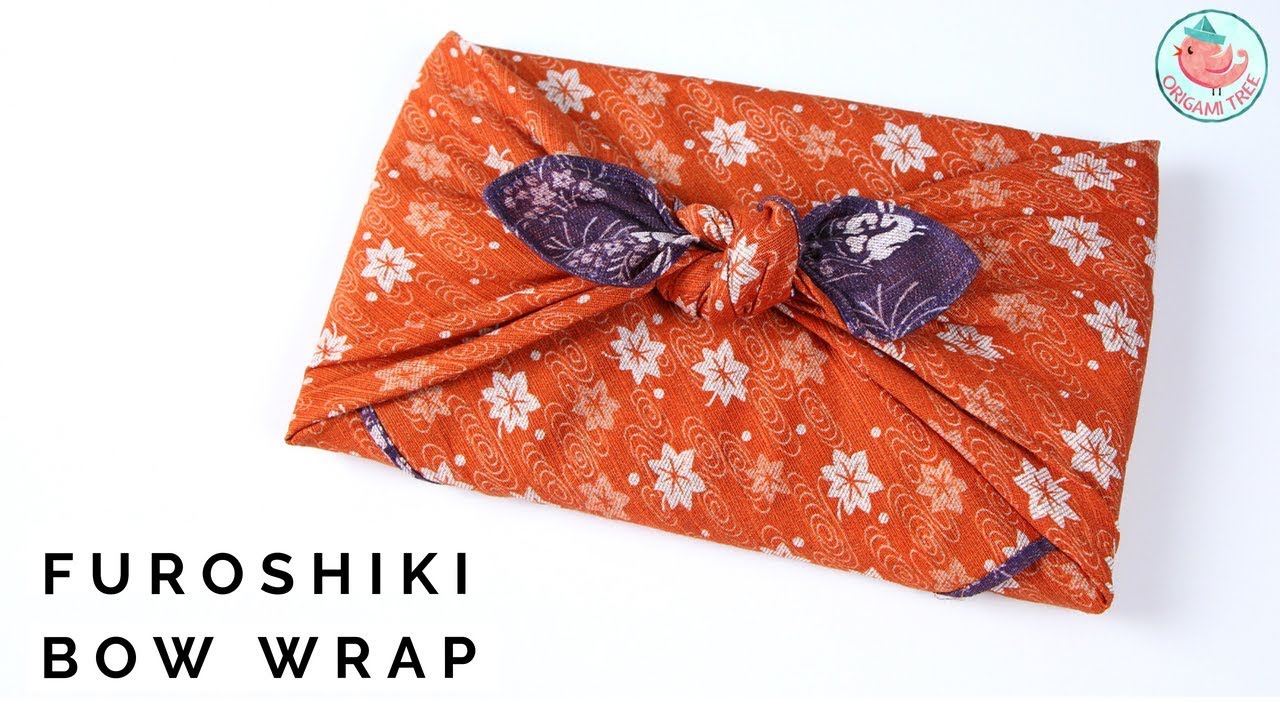The image features a wrapped item centrally placed against a pure white background, casting a slight shadow. The item is wrapped using a Furoshiki Bow Wrap technique, indicated by the text "Furoshiki Bow Wrap" in the lower left corner. The main fabric is a red or red-orange cloth decorated with a diagonal pattern of white flowers or leaves. The wrap is not quite twice as wide as it is tall and appears very flat. There is also some visible purple fabric, possibly indicating a two-sided handkerchief or multiple fabrics. In the upper right corner, a small circular emblem contains the text "Origami Tree" arcing along its circumference. Within the circle is a pink bird facing left, donning a paper origami hat.